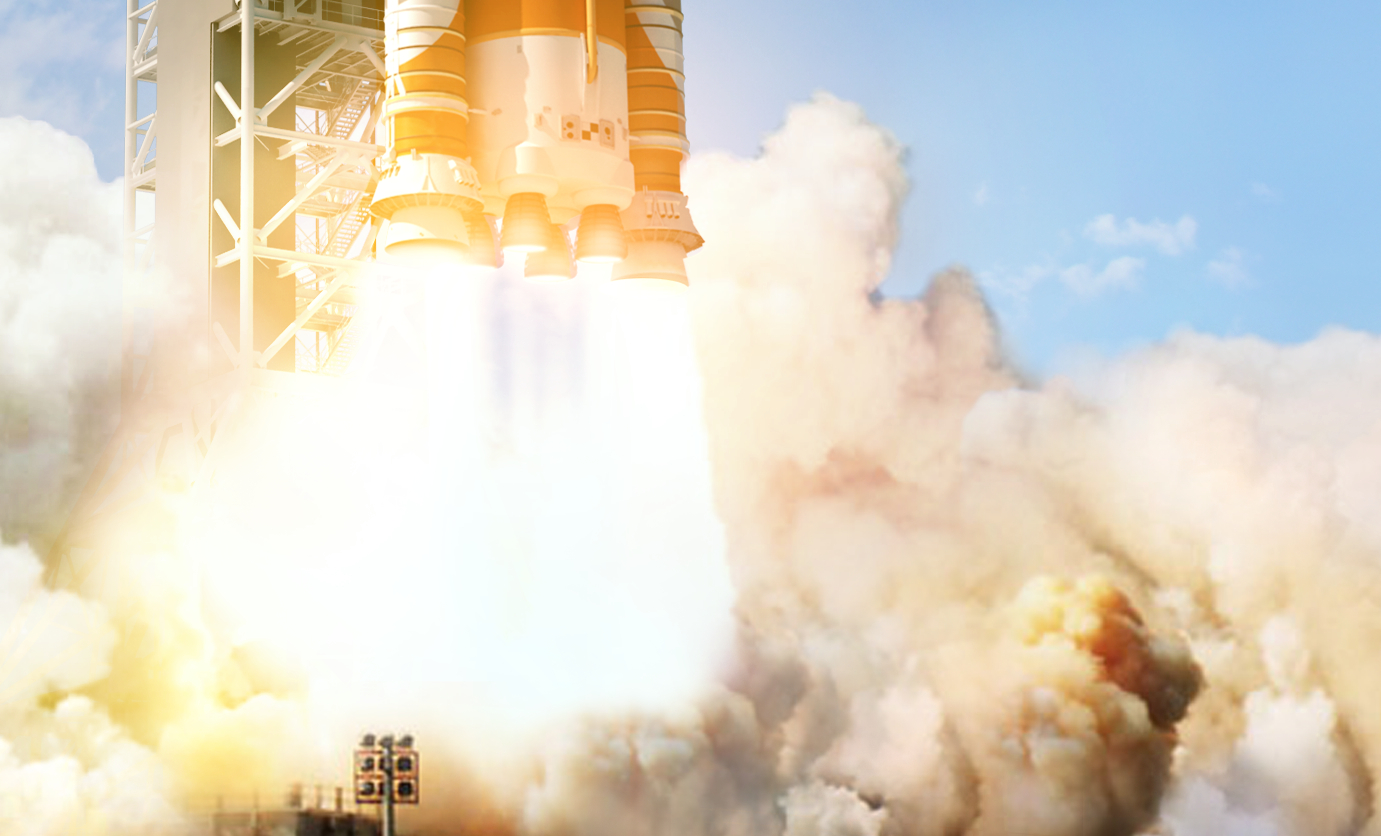This photograph captures the dramatic moment of a Saturn V rocket launch during a clear day. At the bottom of the image, large, swirling clouds of smoke, predominantly off-white with tinges of gray, yellow, and dark orange, billow majestically. A vivid, bright white light—indicative of the fiery exhaust from the rocket—pierces through the smoke on the left side. Rising above this fiery plume, the bottom sections of the imposing Saturn V rocket are visible, showcasing classic orange and white hues as it propels upward. Adjacent to the rocket, on the left, stands a tall metal tower with winding stairs, crucial for supporting the rocket and allowing access. The bright blue sky, unobstructed by any clouds, peeks through at the top right and left corners of the image, contrasting sharply with the dense, colorful smoke that dominates much of the scene.